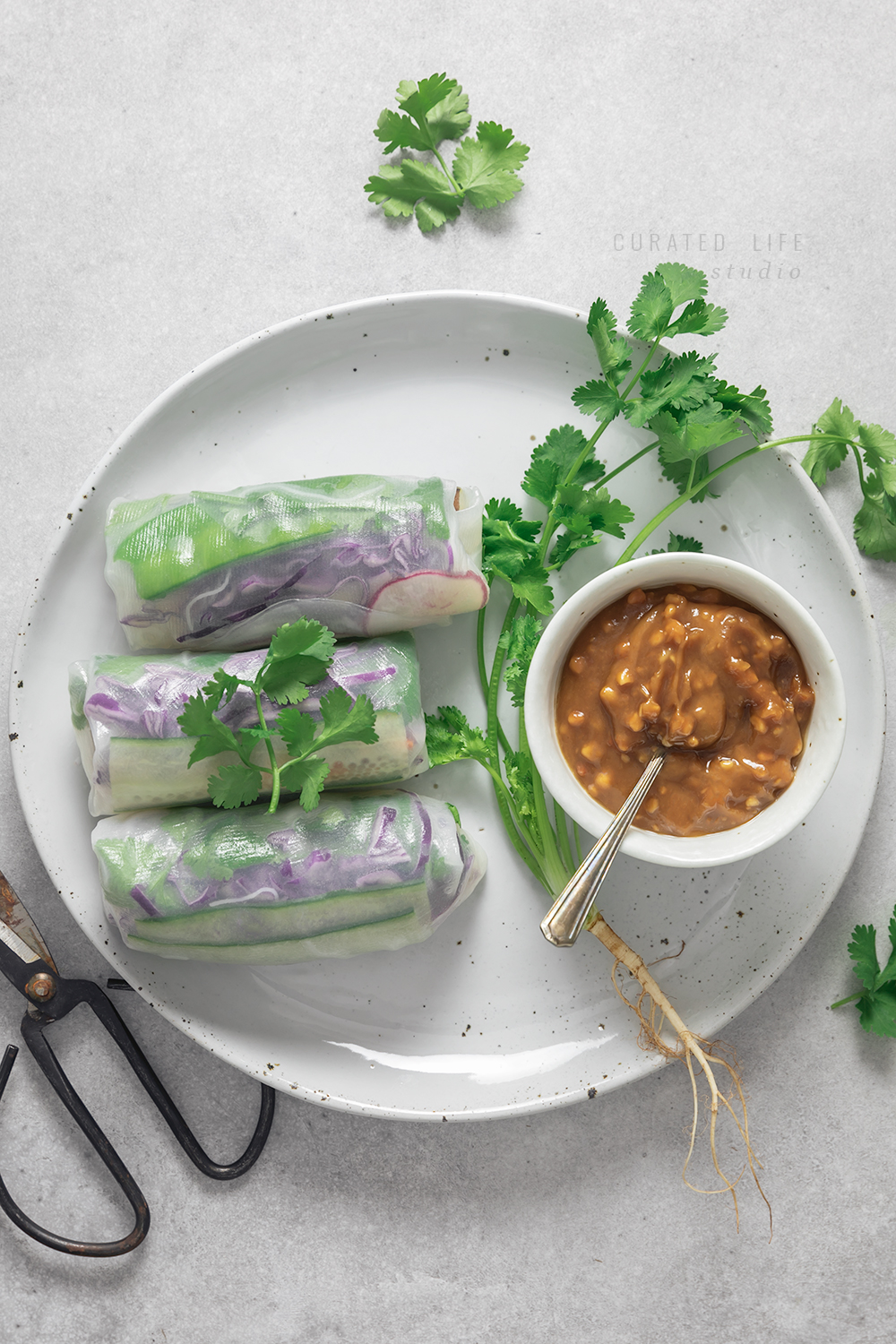This photograph depicts a close-up view of a white plate, adorned with tiny black specks, set against a very light gray background. The plate features three translucent spring rolls, stacked to one side, revealing a medley of colorful vegetables inside, including cabbage, radish, cucumber slices, peas, and rice. These fresh rolls are garnished with cilantro, with some leaves scattered both on and around them. Adjacent to the rolls, there is a small circular bowl containing a creamy brown bean or peanut sauce with a silver spoon emerging from it. A stalk of parsley with roots is also present, adding a rustic touch. Interestingly, a pair of metal-handled scissors, slightly rusty, rests by the plate, possibly included for cutting the herbs. The image is noted to be vertically oriented and features a watermark in the top right corner that reads "curated life."